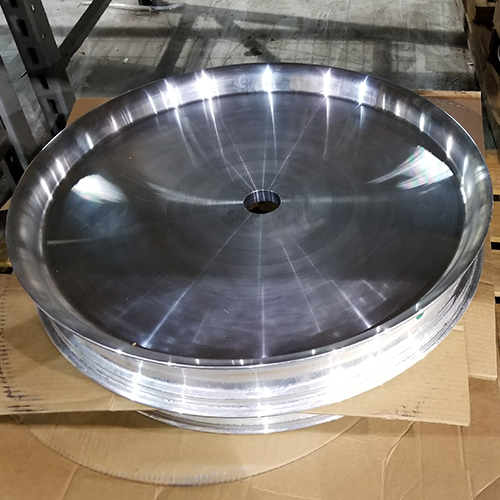In the image, we see a close-up of a shiny, metallic, silver dish-like item, which appears to be the insert of a tire wheel without the actual tire. The bright silver outer rim and the polished, gray center, complete with an open, round hole, reflect light, possibly from an overhead source. This item rests on several pieces of cardboard, likely its original packaging, and is placed on a concrete floor. In the background, a gray porch with metal or wooden bars intersecting both horizontally and vertically can be seen, along with shadows of other metal structures, possibly a ladder, casting across the scene.